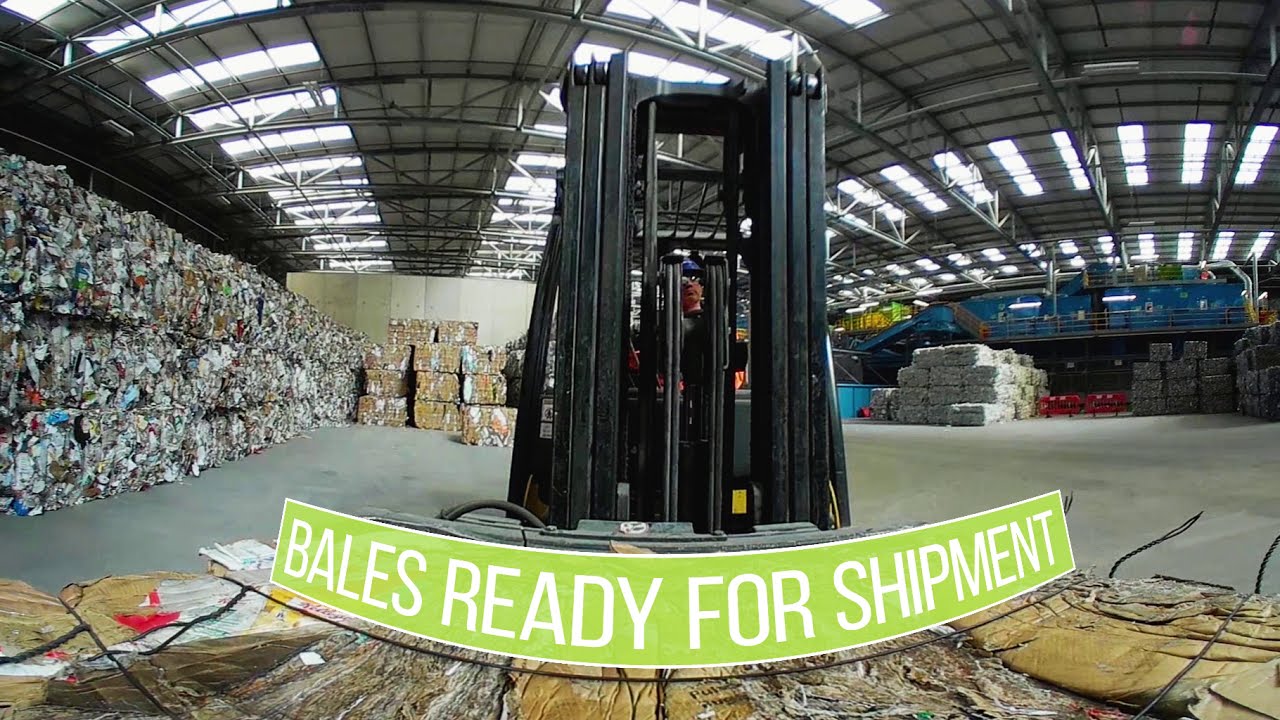The image depicts the interior of a warehouse with a horizontal sign at the center that reads "Bales ready for shipment" in neon green with white text. The sign is positioned just below large black machinery, likely a forklift, which occupies the central part of the image, indicating that the photograph was taken from the perspective of the forklift's camera. Stacked on both the left and right sides are three layers of recycling material, predominantly bundles of paper bales, forming large, brick-like towers. The warehouse's ceiling is visible at the top of the image, illuminated by large lights and natural sunlight filtering through sunlights. The overall setting is an organized expanse, prepared for shipment of the recycled materials.